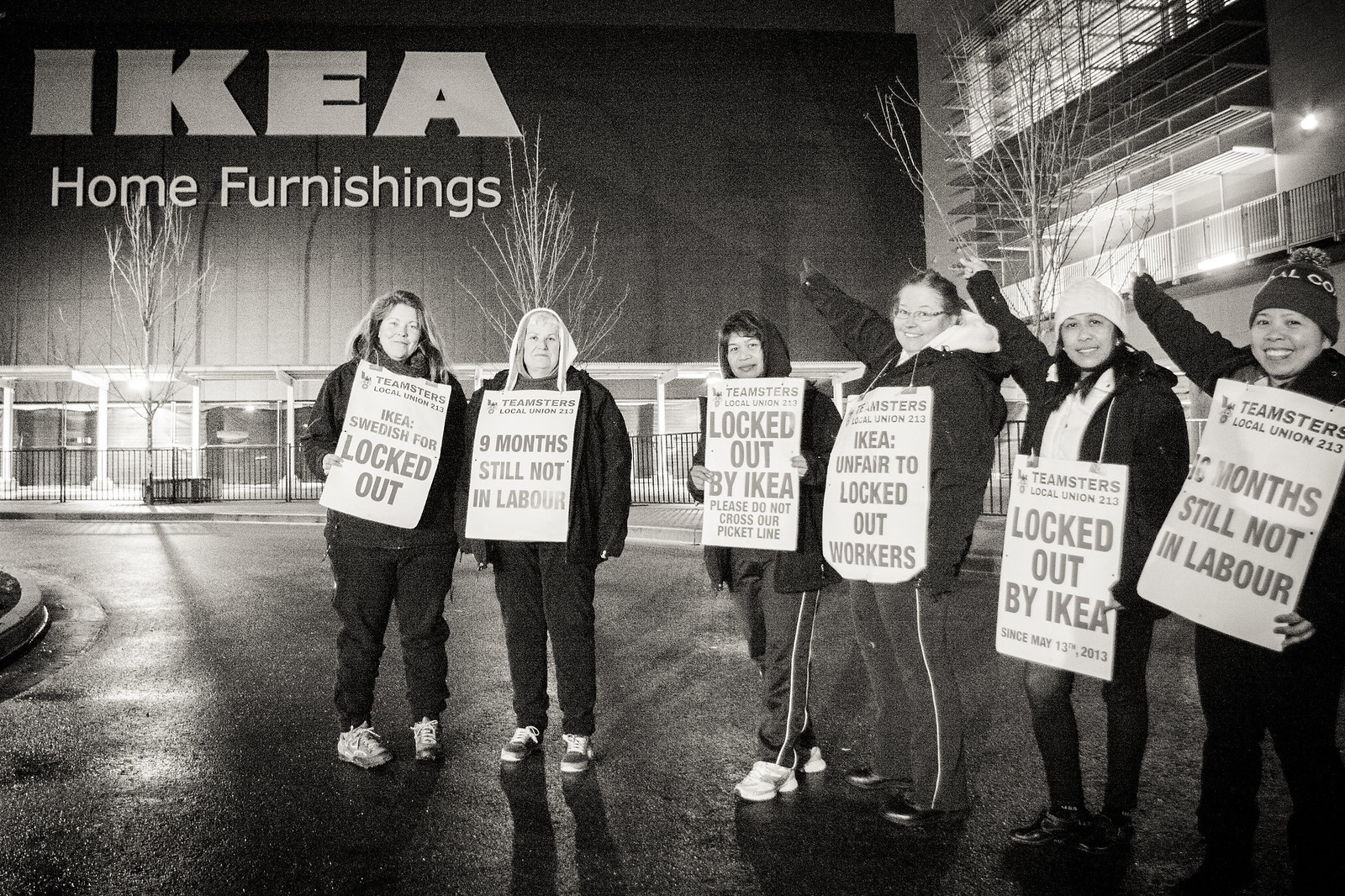In this compelling black-and-white image, six determined women stand resolutely outside an IKEA home furnishings store, with the store's signage visible in the top left corner. Bundled up in jackets, hoodies, and some wearing hats against the cold, these members of the Teamsters Local Union 213 are engaged in a strike. Their faces express resolve as they hold up protest signs that read "IKEA, Swedish for locked out," "Nine months, still not in labor," "Locked out by IKEA, please do not cross our picket line," "IKEA, unfair to locked out workers," and "Ten months, still not in labor." The stark contrast of the black-and-white photo highlights both their struggle and their unwavering solidarity in the face of adversity.